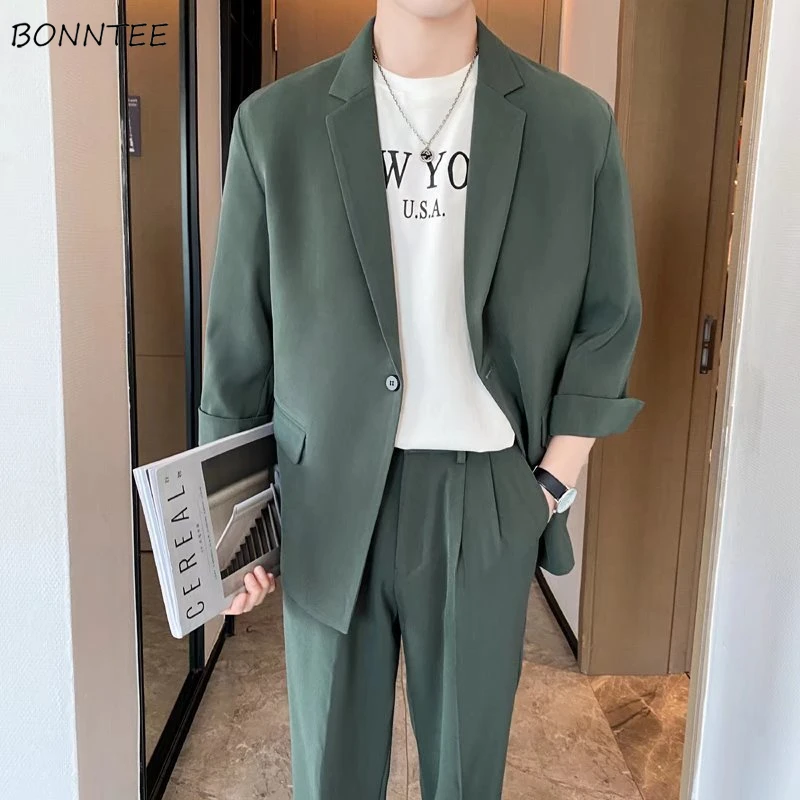In the image, a young male model is showcasing a gray suit ensemble, consisting of a suit jacket and pleated pants. He pairs the outfit with a white t-shirt emblazoned with the letters "W-Y-O" across the chest and "U.S.A." below it. The suit jacket's sleeves are stylishly rolled up, revealing a wristwatch on his left wrist, and his left hand is casually tucked into his pocket. A silver chain with a small pendant falls to the "Y" on his t-shirt. In his right hand, the man holds a magazine titled "Cereal," which features an image of stairs on its cover. The model stands in a neutral-toned hallway with tan tile flooring. Behind him are a series of brown doors, and a mirror is mounted on the left wall. In the upper left corner of the image, the brand name "BONNTEE" is displayed in bold, black uppercase letters. The overall setting and wardrobe suggest a stylish clothing brand advertisement.